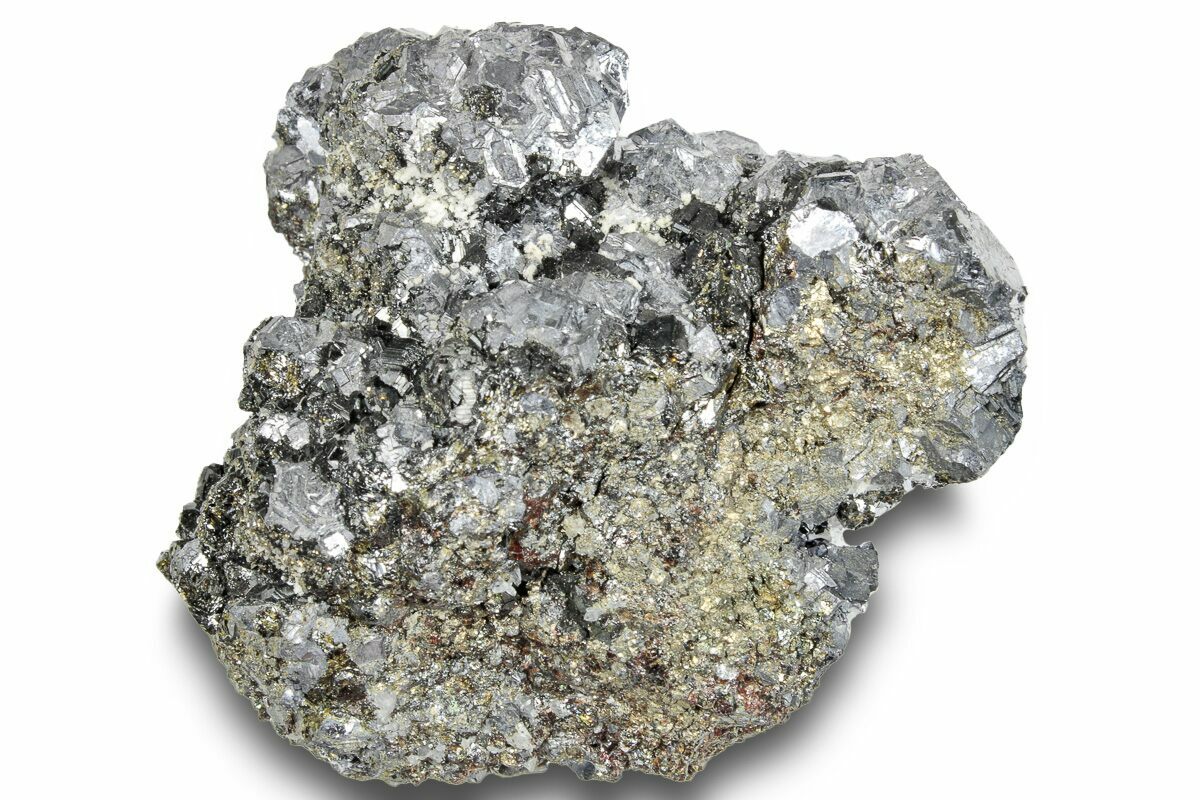The image features a detailed close-up photograph of a rough, irregularly-shaped mineral rock set against a stark white background. The rock casts a shadow on the bottom, emphasizing its three-dimensional form. Predominantly gray in body, the rock showcases an array of colors including white, yellow, orange, and hints of red, giving it a vibrant, multi-faceted appearance. The base and bottom left corner of the rock display a yellowish hue, while the top transitions to a more silvery or whitish-gray, resembling silver crystals or possibly fool’s gold. The texture of the rock varies, with rough, small, goldish, and coppery sections at the bottom, transitioning to more cubic, salt-like, and clearer or silver-toned surfaces along the top. The top ridge is especially distinguished, appearing almost transparent under the light.